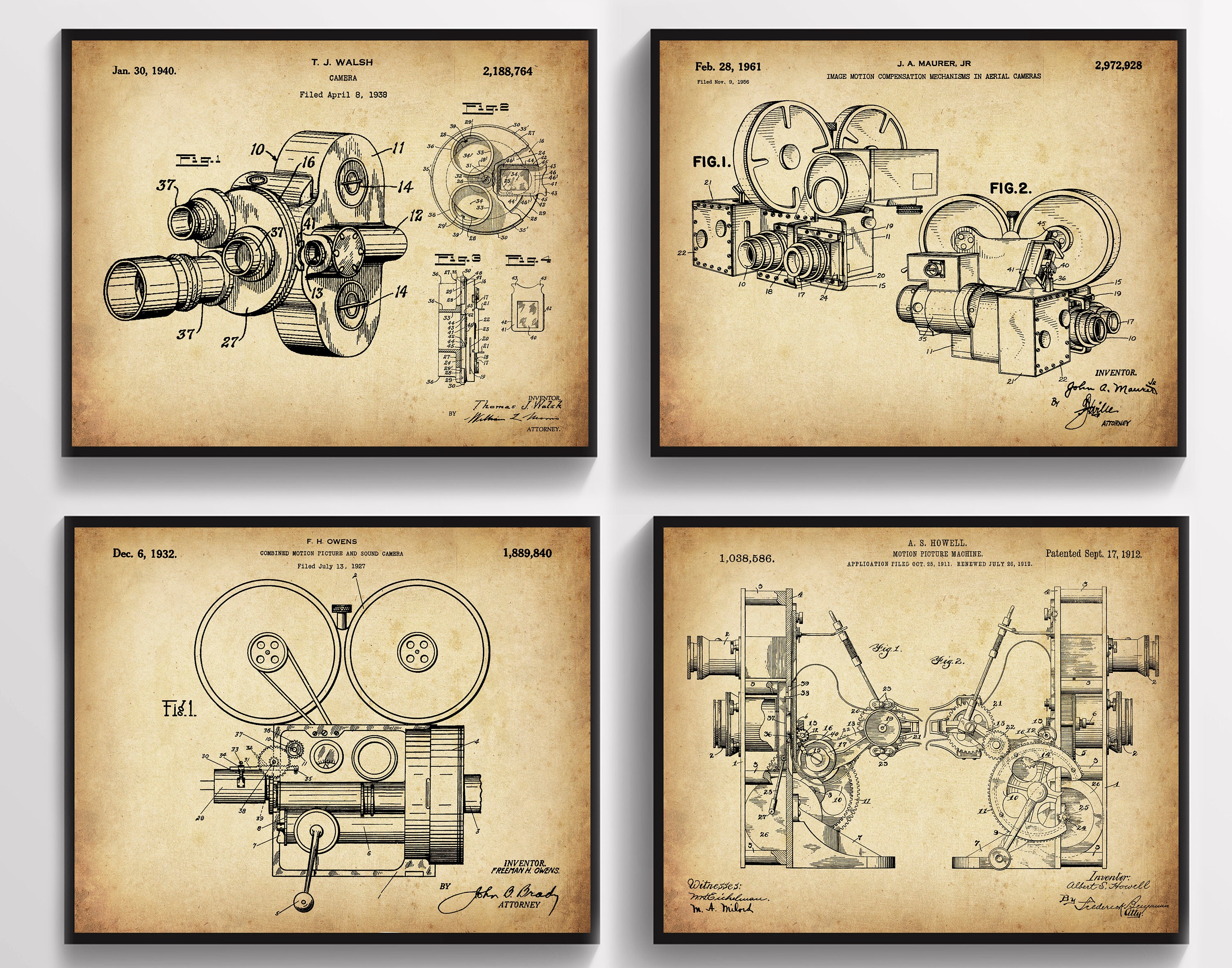This image showcases a series of four symmetrically arranged, framed diagrams of film cameras, meticulously illustrated with intricate details. Each image is set against a parchment-colored background and has a dark brown border, emphasizing their vintage and technical nature. The top left diagram features a camera slightly angled with various parts labeled, showing the lens facing left and the body centered. The top right diagram presents two different camera views, each with exploded views and detailed annotations. The bottom left image provides a side view of the camera, displaying the canisters on top and the barrel below, showing internal components with the lens facing left. The bottom right diagram depicts the front view of the camera, divided in half with its components separated and labeled. Each image resembles patent drawings, complete with dates and patent numbers from different historical periods, ranging from the early 19th century to the mid-20th century, illustrating the evolution of camera design over time.